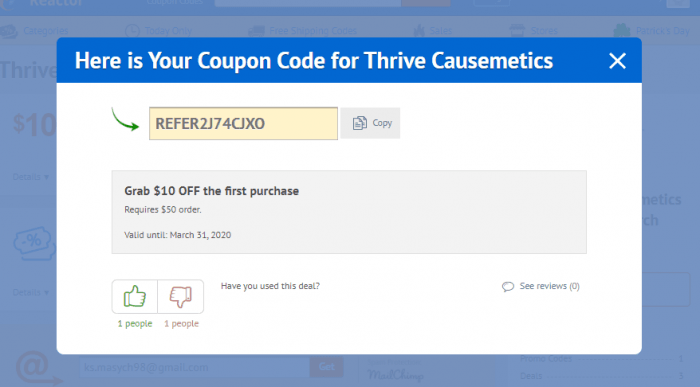Caption:
"Grab $10 off your first purchase with a minimum order of $15! This offer is valid until March 31st, 2020. To redeem, use the provided code and send it through. User reviews show varying opinions, with a green thumbs-up from 1 person and a red thumbs-down from another. Take advantage of free shipping codes available today only. Potential categories include Patrick's Day, special deals from Thrive, and other text-related offers. A significant aspect appears to be a square icon at the center of the image, possibly indicating an important link or action button. Check out Mad Mailchimp for more diverse text deals and offers."